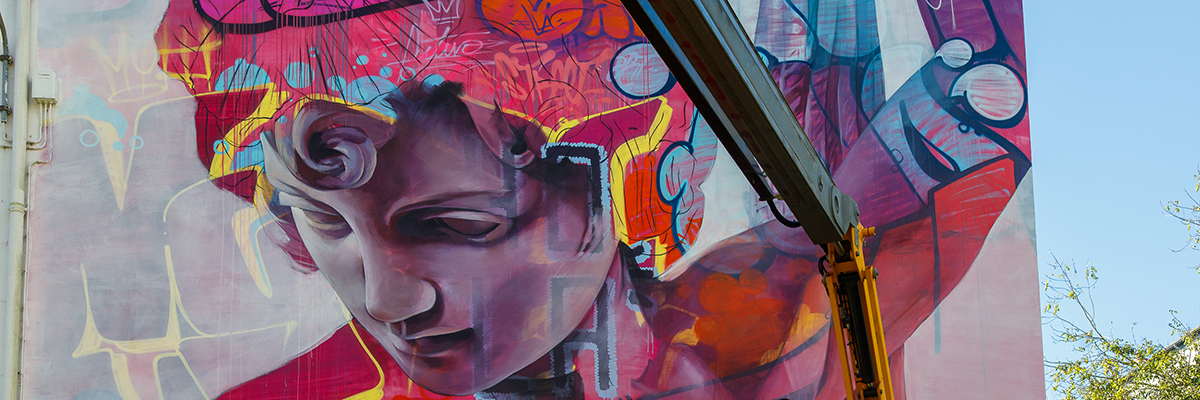The image is a vibrant, landscape-oriented photograph featuring a mural painted on a grayish-creme wall. The right-hand border showcases a light blue sky dotted with thin branches bearing green leaves, hinting at an outdoor setting. Intriguingly, the scene includes a mechanical crane arm, painted in yellow and black, likely used for accessing higher parts of the mural. The central focus is on an abstract, graffiti-styled portrait of a person, seemingly a boy, depicted with striking detail. His face, rendered in a purplish stone hue, carries the serene expression reminiscent of a Greek statue, with curly hair flowing into a cascade of vivid reds, yellows, maroons, and blues. This colorful extravagance extends to his shoulders and left arm, creating a dynamic contrast against the muted background. On the bottom right, part of what appears to be a white roof is visible, adding subtle architectural context to the vibrant display.